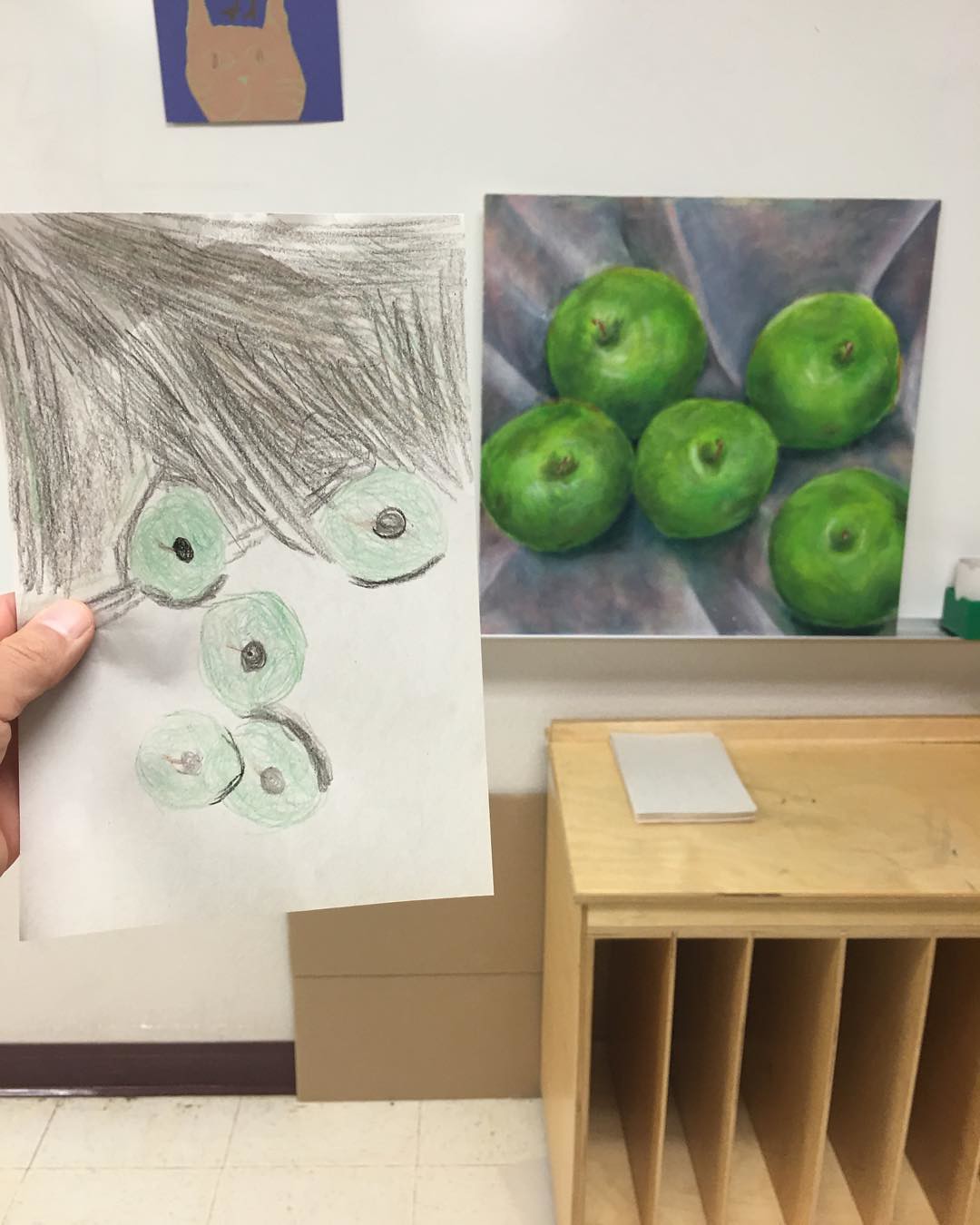In the photograph, a hand emerges from the left side, holding a child's drawing of five green apples rendered with green crayon. The apples are encircled with black edges, and the upper third of the drawing is scribbled with black crayon. This drawing is held up against the backdrop of a room featuring a simple tan desk with vertical slots underneath, ideal for storing large items or paintings. On the desk, there sits a notepad and a folded corrugated box pushed against the wall. The room is finished with simple linoleum tiles and baseboards. Above the desk, two images adorn the cream-colored wall: a children's drawing of a brown cat face on a blue background, and a proper painting of five bright green apples in what appears to be a silver bowl, set against a gray fabric backdrop with light and dark folds creating shadow and depth.